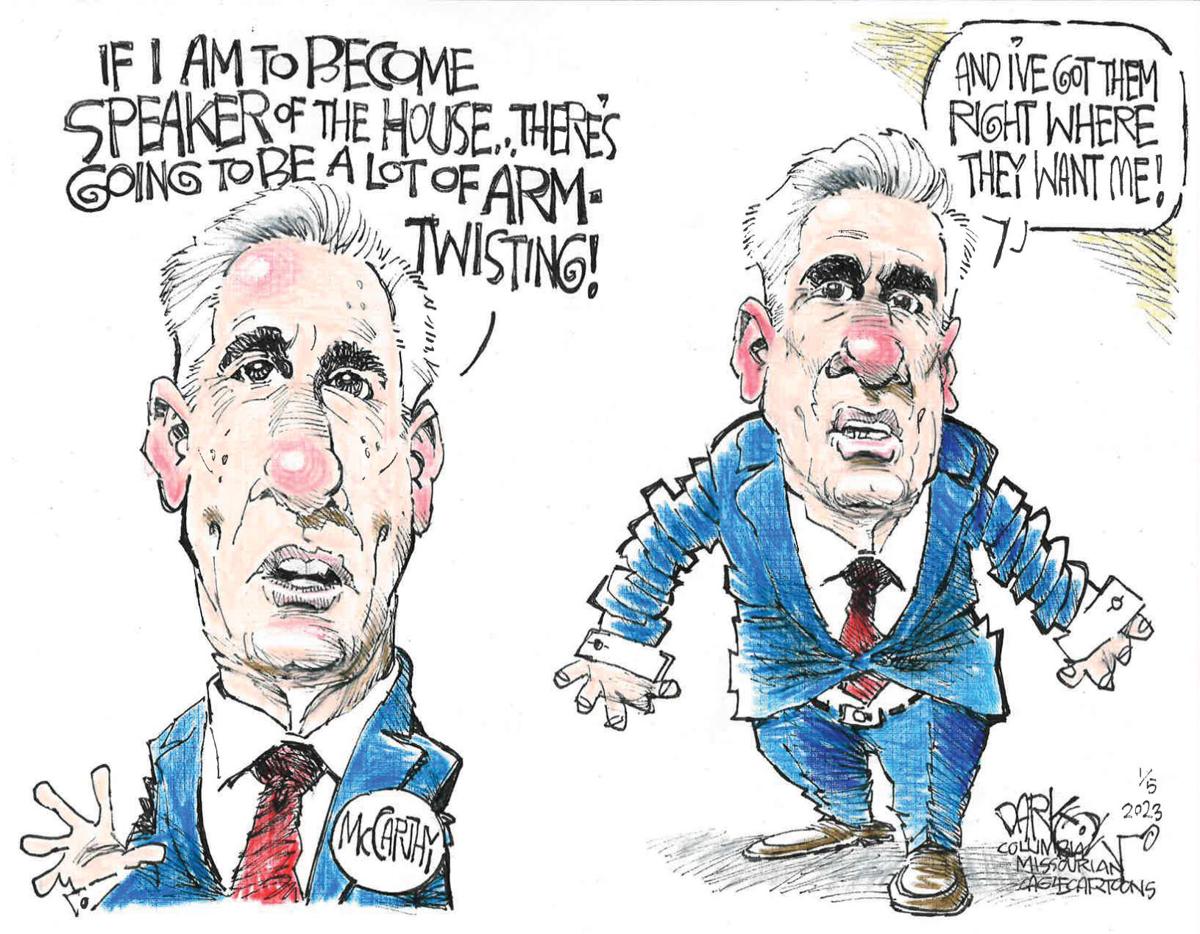The image is a political cartoon in a caricature style featuring Kevin McCarthy. It contains two panels set indoors. The left panel is a head-and-shoulders shot of McCarthy dressed in a blue suit, white shirt, and red tie, with his right hand held open. He has distinctive white hair, a red nose, red eyes, and red ears. His mouth is open as he looks directly at the camera and says, "If I am to become Speaker of the House, there's going to be a lot of arm twisting."

The right panel shows a full-body view of McCarthy, still in the blue suit which is bulging at his waist, emphasizing the strain on the button. He wears a belt and brown shoes, and his hands are stretched out. His red nose and ears are consistent, and in this panel, he declares, "And I've got them right where they want me." The bottom of the cartoon includes the text: "D-A-R-K, Columbia, Missourian, C-A-G-F, cartoons, 1/5/2023." The overall scene captures the essence of political satire with exaggerated features and expressions.